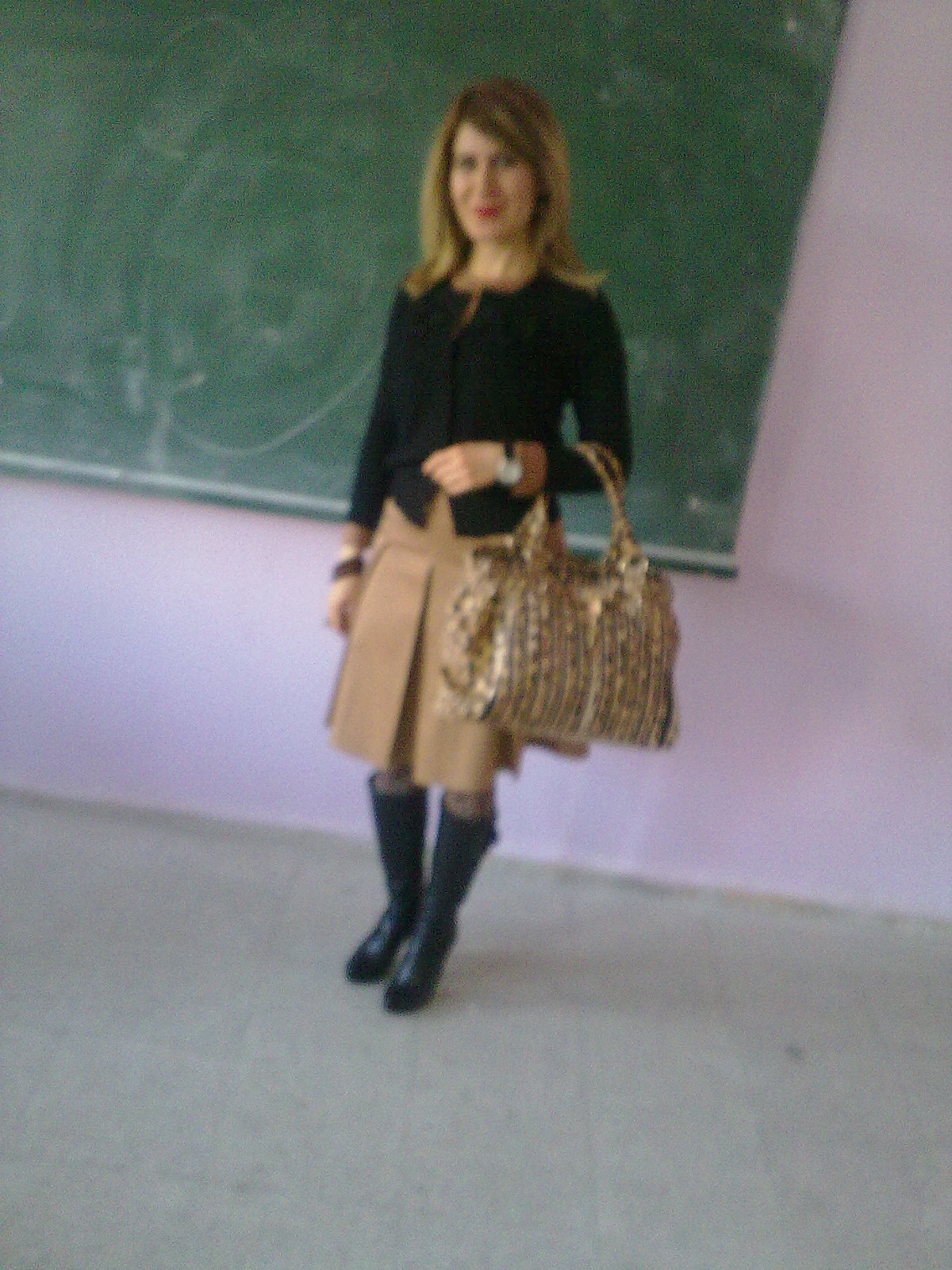A blurry photograph captures a smiling blonde woman standing in what appears to be a classroom with lavender pinkish walls. Behind her, a green chalkboard with faintly erased circles is mounted on the wall. The floor is covered in plain, gray ceramic tiles. She is dressed in a black, buttoned-up cardigan sweater paired with a beige, knee-length pleated wool skirt and knee-high black boots with heels. Her bright red lipstick adds a pop of color to her look. She wears a black watch and a bracelet on her left wrist. Draped over her arm is a large, gold shimmery purse with black handles.